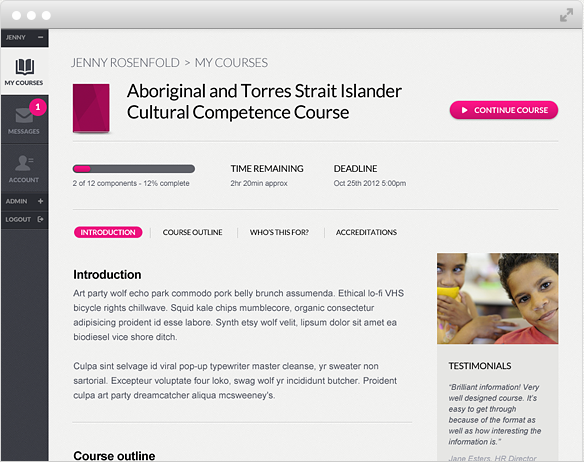This screenshot displays a webpage showing the progress overview for a user's online course. At the top, the page is labeled with "Jenny Rosenfold," and an arrow points towards the "My Courses" section, indicating that the user is currently on the "My Courses" page. The specific course in view is the "Aboriginal and Torres Strait Islander Cultural Competence Course." 

Central to the screen, there is a prominent pink button labeled "Continue Course," adorned with a white arrow pointing to the right. Below this, progress statistics reveal that the user has completed 2 out of the 12 course components, equating to 12% completion. The remaining time for course completion stands at approximately 2 hours and 20 minutes, and the deadline is specified as 5:00 PM on October 25th, 2012.

Further details include sections titled "Course Outline," "Who's this for," and "Accreditations." The "Course Outline" lists different components such as "Introduction," "Art Party," "Wolf Echo Park," "Commodore," "Park Belly," and "Brussels Assembly." 

A user comment praises the course, describing it as brilliantly informative, well-designed, and easy to navigate due to its engaging format and interesting content.